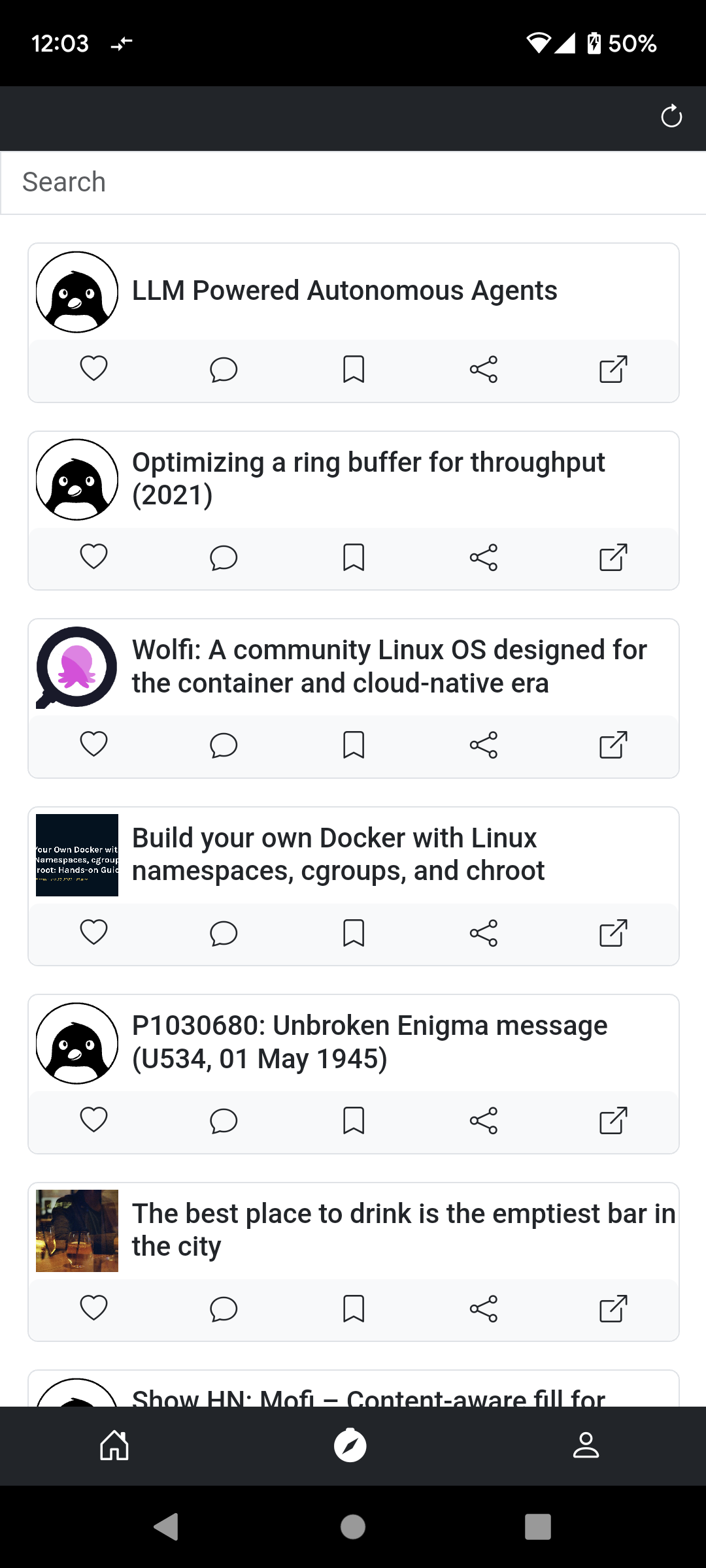This is a screenshot taken from a smartphone, featuring a user interface with a black border. In the top left corner, there is a timestamp indicating 12:03, accompanied by left-facing and right-facing arrows stacked above each other. On the top right, the icons for Wi-Fi and battery status are visible, with the battery level shown at 50%.

Beneath these icons, there is a refresh arrow followed by a search bar. Below the search bar, the screen displays a list of what appear to be social media posts. Each post includes options to like, comment, bookmark, share, or close it.

The first post features a photograph of a penguin, with the caption “LLM-powered anonymous agents.” Directly below that is another post from the same user, represented by the penguin photo again, with the text, “Optimizing a ring buffer for throughput 2021.”

The third post features an image of a squid inside a magnifying glass and reads, “Wolfie, a community Linux OS designed for container and cloud-native error.” The following post has a black box with white text that is unreadable, titled, “Build your own Docker with Linux namespaces, cgroups, and CRUT.”

Further down, there’s another post using the penguin photograph, this time captioned, “P1030680, unbroken enigma message (U534), 04 May 1945.” 

The next post mentions, "The best place to drink is the emptiest bar in the city. I agree," but the details of the accompanying image are unclear as it appears to be a square or some unclear shape.

The final visible post mentions “Show agent Mophie, content-aware filled four,” but the text is cut off at the end.

At the bottom of the screen, the black border reappears, containing icons for home, user profile, and an unknown middle icon. Below these icons, there are additional controls including a left-facing arrow, a home button, and a stop button.